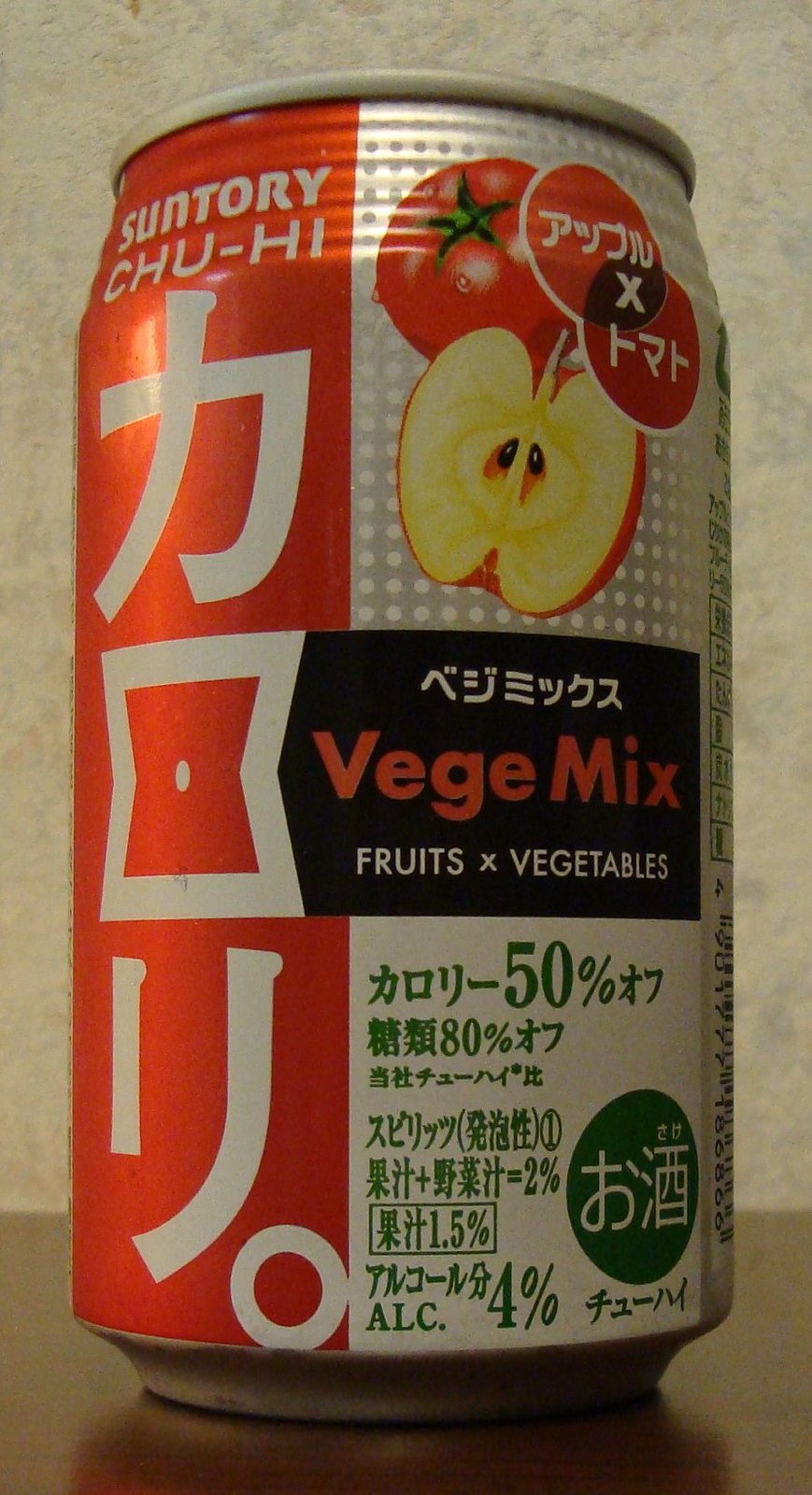This is a detailed color photograph featuring a can of Japanese soda. The left side of the can prominently displays the brand "Suntory," written both in English and Japanese katakana (C-H-U HI). Below this branding, large white katakana letters spell out "KALORI," which translates to "calorie." 

To the right, the can transitions into a silver background with a distinctive black label. Above the writing, there is a vivid photograph of a fresh tomato adorned with water droplets, alongside a halved apple that reveals its yellowish-white flesh and two black seeds.

At the top of the can, two small circles contain Japanese katakana characters that translate to "apple" and "tomato." Underneath the photograph and within the black label, the product name "VEGEMIX" is written in striking red letters, followed by the phrase "Fruits and Vegetables" in English. 

Additional Japanese text is present, which indicates that this beverage contains 4% alcohol. The overall design effectively communicates a blend of fruit and vegetable flavors, augmented by clear branding and appealing imagery.